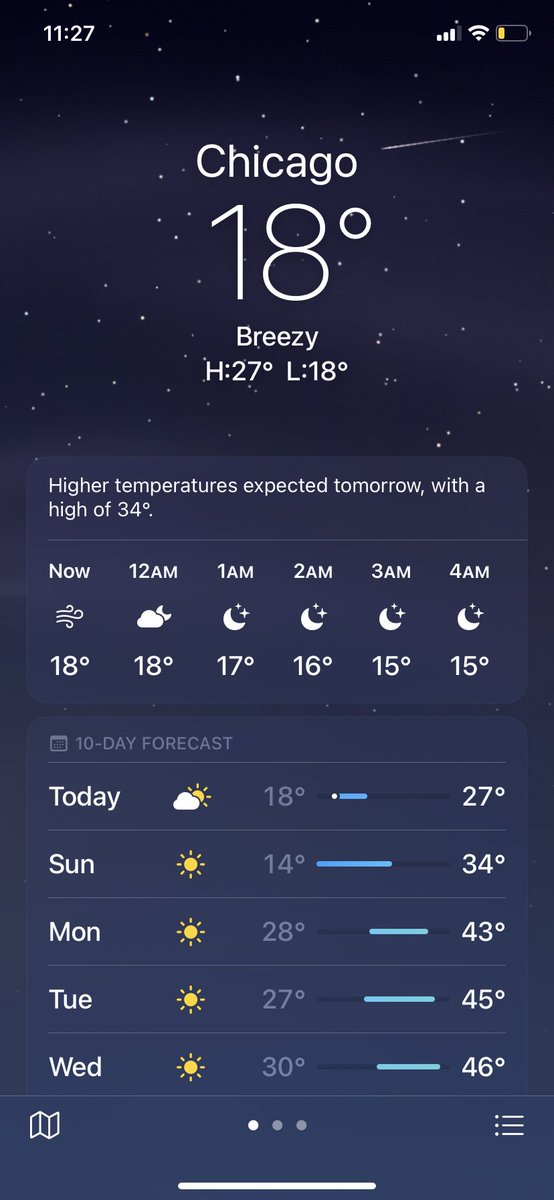The image is a detailed screenshot of a weather app displayed on a mobile device. The background is a dark night sky dotted with white stars, contributing to the overall theme.

### Top Section:
- **Time and Status Indicators:** 
  - At the very top left corner, the time is displayed in white as "11:27".
  - The top right corner features standard status indicators: Wi-Fi signal strength and battery level, marked at 15% with a yellow fill.

### Main Weather Display:
- **City and Current Temperature:** 
  - The city "Chicago" is prominently displayed in white at the center-top.
  - Below the city name, the current temperature reads "18°" and is accompanied by the description "Breezy".
  - The high and low temperatures for the day are indicated as "H: 27°" and "L: 18°".

### Weather Update Box:
- **Weather Forecast:**
  - A blue rectangular box features a weather update at the top, stating in white, "Higher temperatures expected tomorrow with a high of 34°".
  - Below this update, a thin gray separator line is present.
  - **Hourly Forecast:**
    - The leftmost column displays "Now" with a wind symbol and "18°".
    - Successive columns show:
      - "12 a.m." with a cloud and crescent moon icon, "18°".
      - "1 a.m." with a cloud and two stars icon, "17°".
      - "2 a.m." with a cloud and two stars icon, "16°".
      - "3 a.m." with the same icon, "15°".
      - "4 a.m." again with the same icon, "15°".

### Extended Forecast Section:
- **10-Day Forecast:**
  - At the top of this longer blue box, a gray heading reads "10-DAY FORECAST" followed by a thin gray separator line.
  - **Daily Forecast:**
    - **Today:** 
      - To the left, marked "Today" with a white cloud and yellow sun icon.
      - Temperature range: "18°" to "27°".
      - Adjacent line chart shows a small blue strip, indicating temperature progression.
    - **Sunday:**
      - Marked "Sun" with a bright yellow sun icon.
      - Temperature range: "14°" to "34°".
      - The line chart is nearly half-filled in blue.
    - **Monday:**
      - Marked "Mon" with a sun icon.
      - Temperature range: "28°" to "43°".
      - The line chart starts in the middle, extending nearly to the end.
    - **Tuesday:**
      - Marked "Tue" with another sun icon.
      - Temperature range: "27°" to "45°".
      - The line chart is slightly longer than Monday's.
    - **Wednesday:**
      - Marked "Wed" with a sun icon.
      - Temperature range: "30°" to "46°".
      - The line chart extends almost to the end, leaving a tiny unfilled segment.

### Bottom Section:
- **Navigation and Menu:**
  - The bottom border typical of mobile apps displays navigation options:
    - To the left, an icon resembling a folded piece of paper.
    - In the middle, a set of three navigation circles; the first is filled in white, the other two are gray.
    - On the far right, a menu icon with three horizontal lines, each with a small circle in front.

This detailed description offers a comprehensive view of the weather app screenshot, covering the various sections and their contents meticulously.